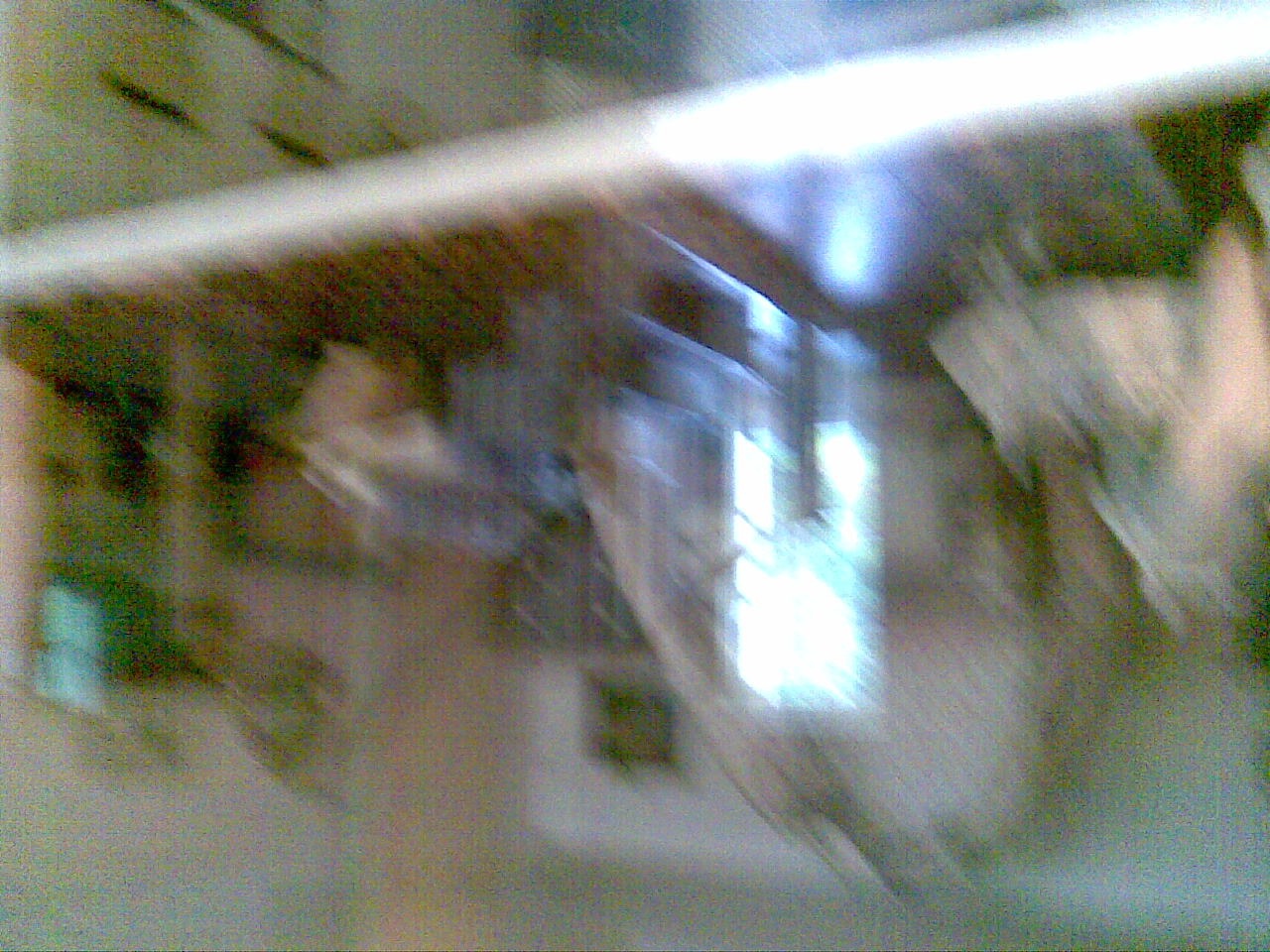A blurry photograph taken during the daytime captures an indoor scene with indeterminate lighting sources, as there is no artificial light visible. The image appears to showcase a shelf, possibly enclosed in glass or Plexiglass, adorned with various small items. There is a bright reflection in the center of the photo, likely caused by a window or door behind the photographer. The overall clarity is poor, making it difficult to discern specific details about the objects on the shelf. The photo is taken in landscape orientation.